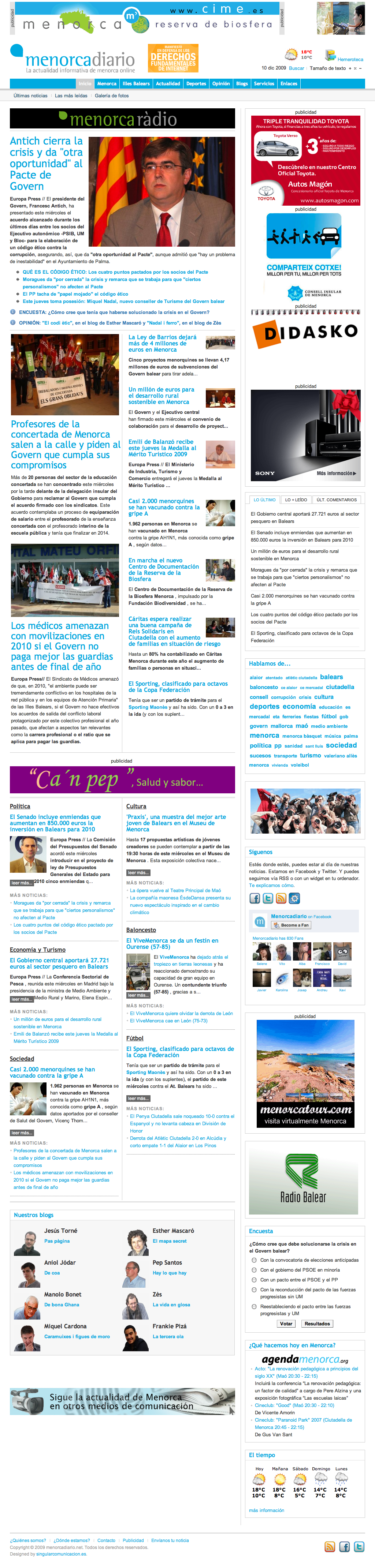The image depicts a very long, thin vertical layout with a predominantly white background. At the very top, it prominently features the heading "Menorca Radio," framed by wide blue and grey lines. Below the heading, there are a couple of logos positioned along with some text that isn't readable due to its small size. Following this section, the first article begins, marked by a dark brown heading. This article includes a photograph of a man clad in a brown suit, red tie, and white shirt, accompanied by additional writing near the image. To the right of this picture, there are two distinct images, one red and one blue. Further down, another smaller image is present. The long layout contains multiple articles written in various colors, including blueprint and black print, with some background sections shaded in purple and green. The bottom segment of the page displays about 20 different hyperlinks, typical of a webpage, suggesting that it is a digital format, possibly a Spanish website given the name "Menorca." On the right-hand side, various advertisements are also visible, contributing to the detailed, text-rich layout of this lengthy digital newsletter-like page.